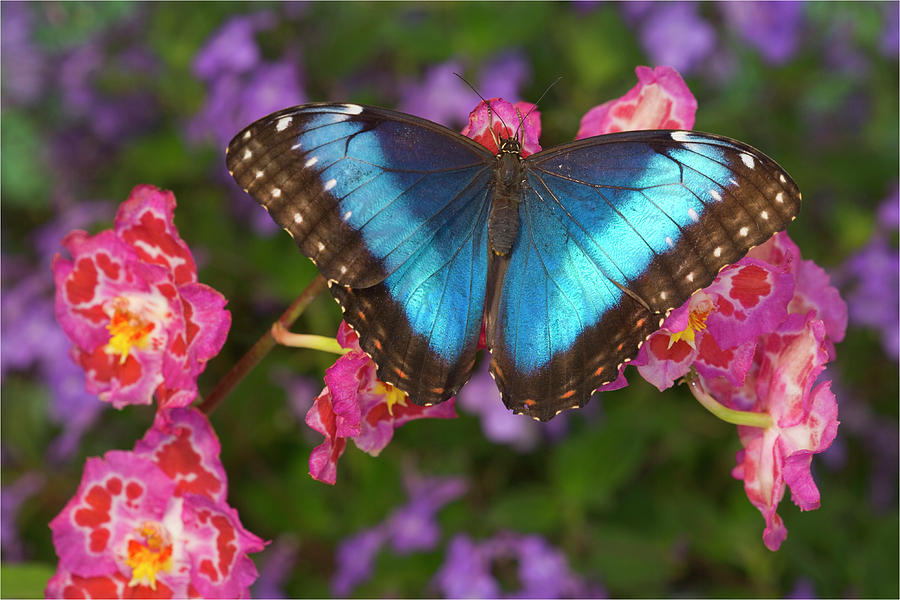The image is a stunning color photograph saturated with vibrant hues. The foreground features an exquisite orchid with half a dozen hot pink flowers adorned with red markings and white outlines. The center of each orchid flower boasts a marigold orange and yellow hue. Perched on one of these striking orchid flowers is a metallic blue butterfly, capturing the viewer's attention. The butterfly's body is black, and its wings display a gradient from dark blue to lighter blue, bordered by black with white and orange spots along the edges. The butterfly's wings are fully open, revealing their intricate patterns. The background is artistically blurred, showcasing green foliage dotted with purple flowers, adding depth and contrast to the vivid foreground. The orchid's brown stem is visible to the left of the butterfly, grounding the composition. Overall, the photograph is a rich tapestry of colors and textures, capturing a moment of natural beauty in extraordinary detail.